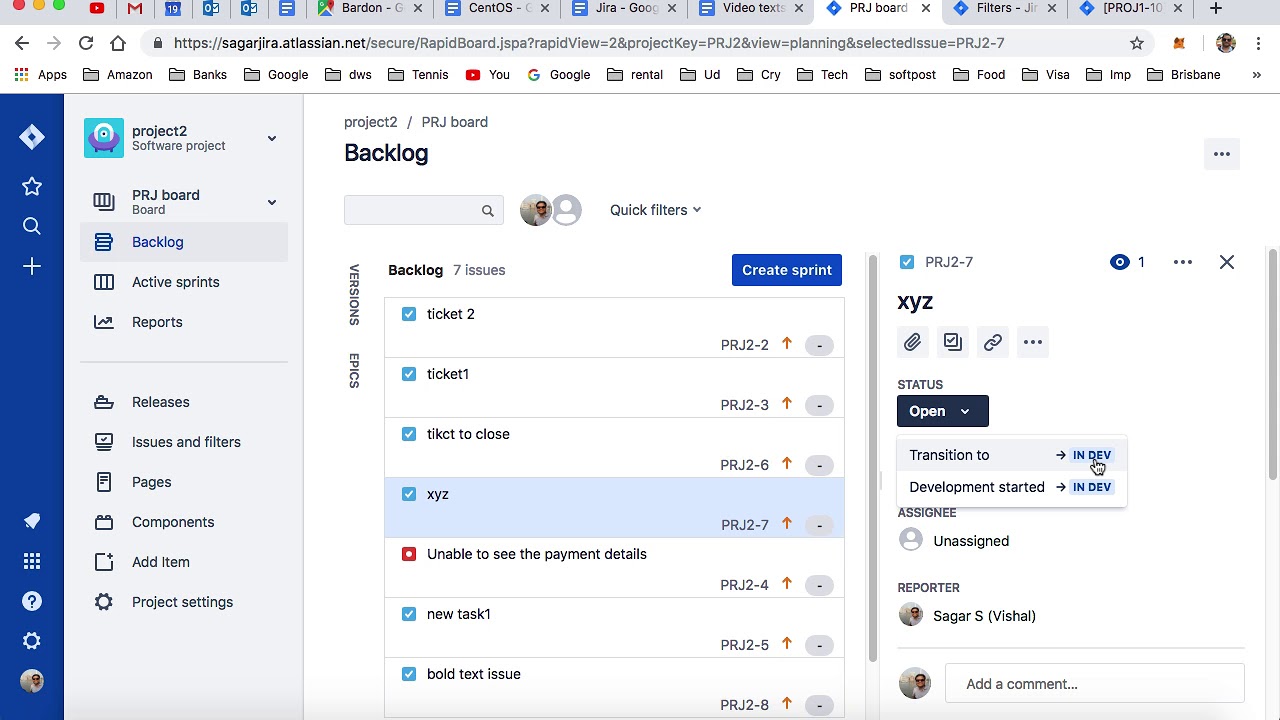A person has numerous browser tabs open on an Apple desktop computer. The familiar red, yellow, and green circles in the top left corner indicate this. Among the open tabs are YouTube, Gmail, Microsoft Outlook, and Google Maps.

The currently active tab features a project management interface. On the left, there is a blue diamond icon with the label "PRJ Board" in black. The main area of the screen has a white background with the title "Project 2/PRJ Board" in bold black text, and a section labeled "Backlog" which lists "7 Issues." A blue button with white text reads "Create Sprint."

Beneath this, various ticket items are detailed:
- "Ticket 2"
- "Ticket 1"
- "Ticket to Close X Y Z"
- "Unable to See the Payment Details"
- "New Task 1"
- "Bold Text Issue"

Each ticket includes status information stating "Open," and suggests transitions such as "Transition to In-Development," "Development Started," and "In-Development." Assessment details show "Assignee: Unassigned" and "Reporter: Sagar (Vishal)."

On the right-hand side of the interface, a navigation menu lists several options: 
- "Project 2"
- "Software Project"
- "PRJ Board"
- "Backlog"
- "Active Sprint"
- "Reports"
- "Releases"
- "Issues and Filters"
- "Pages"
- "Components"
- "Add Item"
- "Project Settings"